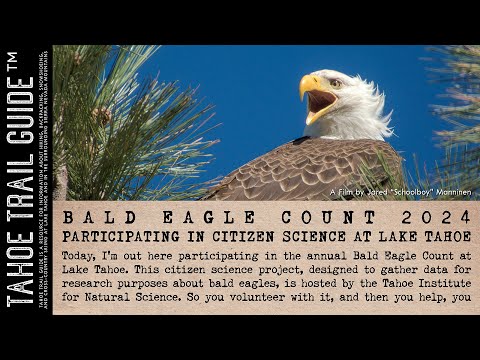This image appears to be a screenshot of a social media or blog article with a completely black background showcasing a citizen science project at Lake Tahoe. At the top left in white text, it reads "Tahoe Trail Guide™" which is vertically aligned. In the center is a vibrant horizontal photograph of a Bald Eagle against a background of green conifer branches and a bright blue sky. The Bald Eagle, with a brown body, white head, and yellow beak, is facing right but turns its head to the left, with its open beak and wind-ruffled feathers highlighted by the sunlight. Below the photograph is an article with a tan background. The headline "BALD EAGLE COUNT 2024" is in all caps, followed by the subheadline "PARTICIPATING IN CITIZEN SCIENCE AT LAKE TAHOE." The first paragraph begins, "Today I am out here participating in the annual Bald Eagle Count at Lake Tahoe. This citizen science project, designed to gather data for research purposes about bald eagles, is hosted by the Tahoe Institute for Natural Science. So you volunteer with it and they help you." The article continues but is cut off. The detailed description highlights the collaborative nature of the project and the role of volunteers in aiding research.